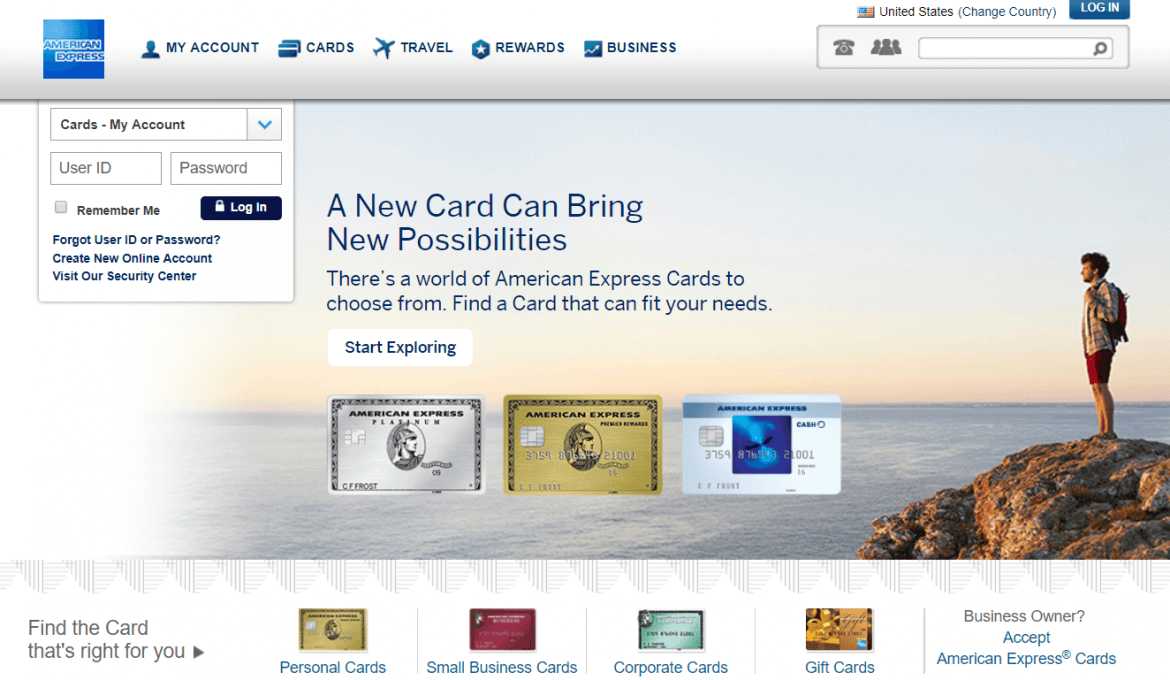The informational page for American Express features a prominent blue square on the left, with "American Express" written inside. On the right side, there's a blue silhouette of a person's head accompanied by various navigation options: "My Account," "Cards," "Travel," "Rewards," and "Business." Below this, there's an option to change the country, marked as "United States," followed by a search bar adjacent to a telephone icon.

To the top right, there's a "Log In" section that includes fields for "User ID" and "Password," along with a clickable "Log In" button. Beneath these fields, there are links for "Forgot User ID or Password," "Create New Online Account," and "Visit Our Security Center."

The center of the page features an image of a man standing on a rock, gazing at the ocean while wearing a backpack, red shorts, and a plaid shirt. Superimposed text reads: "A new card can bring new possibilities. There’s a world of American Express cards to choose from." Below this text, there's a "Start Exploring" button and images of three different American Express cards: one silver, one gold, and one blue.

At the bottom of the page, the tagline "Find the card that’s right for you" appears, along with categories for different types of cards: "Personal Cards," "Small Business Cards," "Corporate Cards," and "Gift Cards."